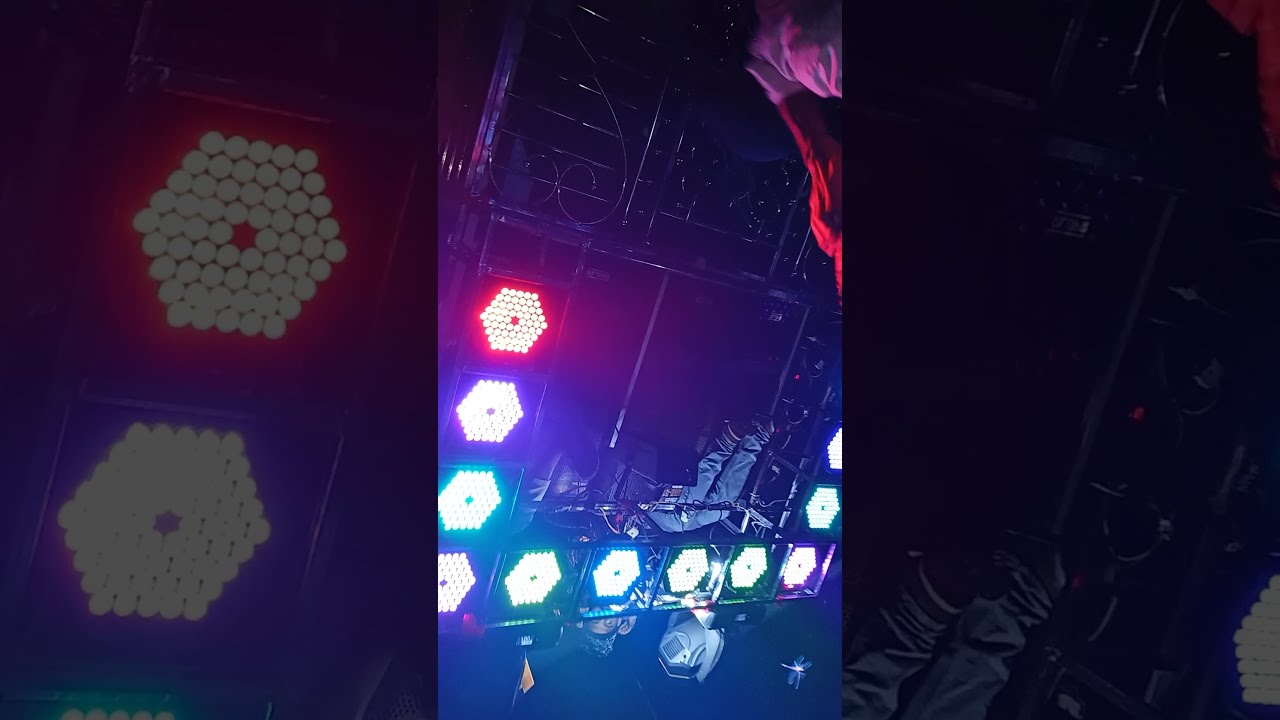The image is a vertically oriented photograph, seemingly taken with a cell phone, featuring an intricate DJ lighting structure. The centerpiece consists of an array of LED lights arranged in a hexagonal pattern, displaying a variety of vibrant colors such as red, yellow, green, blue, pink, teal, and white. The lights form a U-shaped pattern and emit a strong glow, contributing to a dark, concert-like atmosphere. The photograph appears to be inverted, with the camera pointing upwards at what could be either a ceiling or a wall, giving an unclear orientation. The background features the same image but more zoomed in, faded, and blurred, enhancing the central focus. On either side of the main image are vertical sections containing dark, close-up views of the same lighting setup. A man in a red-sleeved shirt is visible near the top right corner of the lighting grid, possibly adjusting the lights or receiving instructions from someone below. There is also a small flag visible on one side and a device, potentially a camera or an additional light, on the other. The overall theme is dark and dramatic, indicative of a stage or stadium setting.